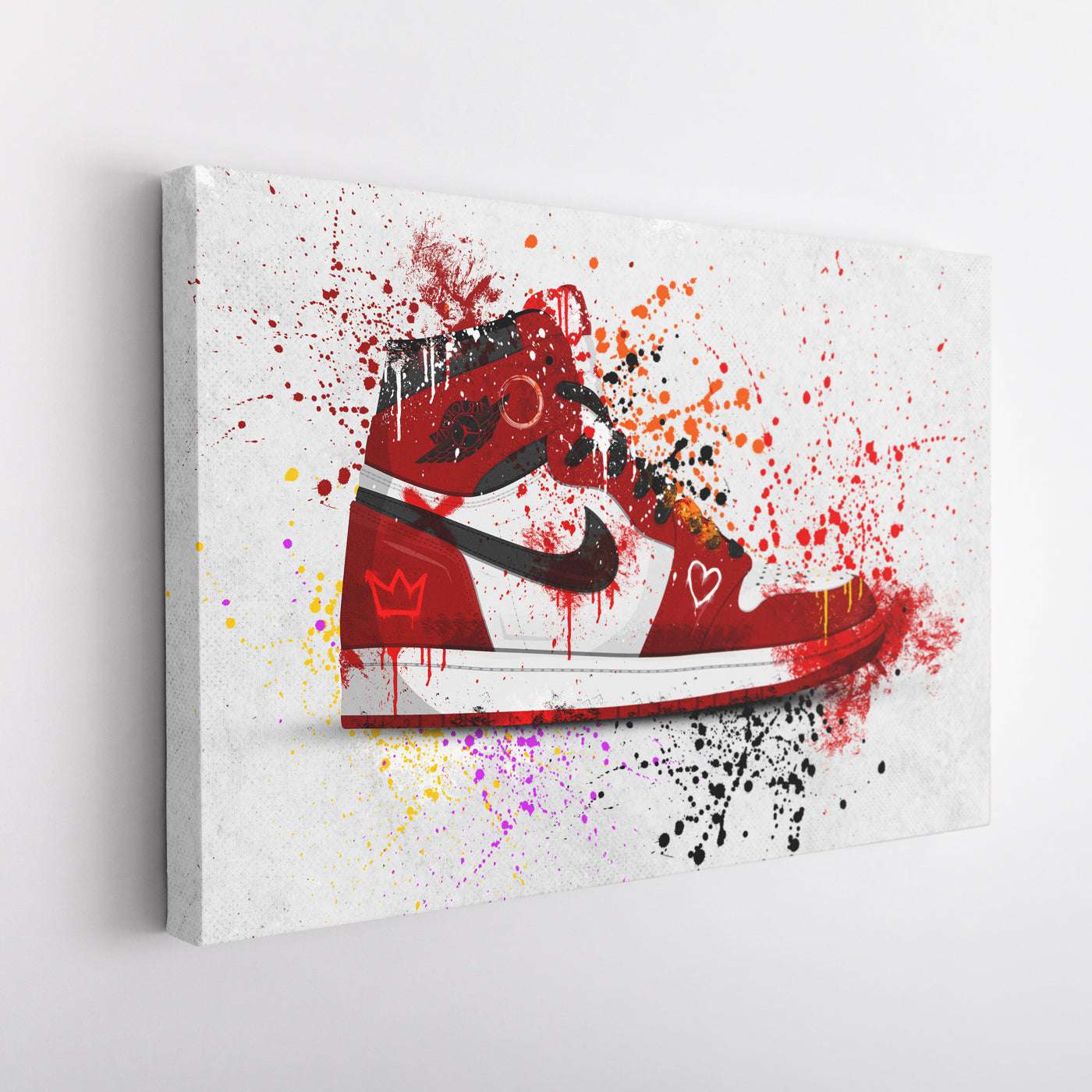This oil painting depicts a highly stylized red Nike sneaker, specifically a high top that resembles an original Nike Air Force One or Nike Air Jordan. The sneaker dominates the canvas, framed in white, and appears viewed from an angle that showcases the left side of the frame. The shoe itself is predominantly red, featuring a black swoosh logo that wraps around the heel and a little white heart spray-painted just before the toe. 

Highlighted details include a light red crown on the dark red heel and laces that are black. The sole of the shoe is primarily white with a red tip at the toe, and the entire shoe is covered in a myriad of paint splatters and drips. These splatters include a variety of colors such as maroon, yellow, pink, orange, and black, giving the appearance that the sneaker was placed amidst a splatter of paints. Additionally, a white ‘O’ can be seen superimposed above the shoe.

The background and frame are stark white, accentuating the vivid hues and dynamic splashes of color emanating from the shoe, making it appear as though it’s bursting with creativity and energy.